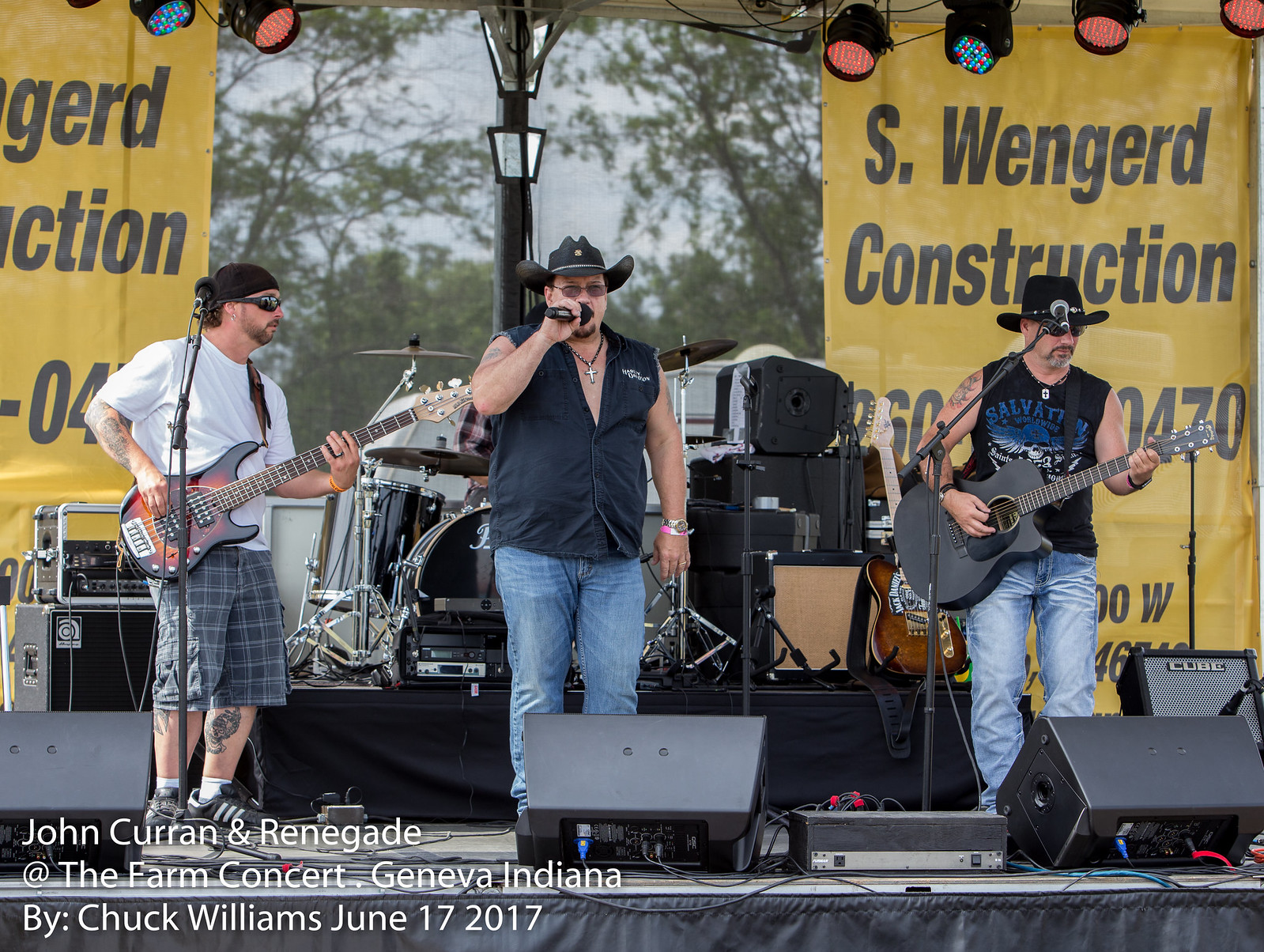The image captures an engaging outdoor concert on a sunny day, featuring the band John Curran and the Renegades at The Farm Concert in Geneva, Indiana, photographed by Chuck Williams on June 17, 2017. Set against a backdrop of clear sky and lush trees, the scene is vibrant with multicolored stage lights strung above. Dominating the stage are three band members: on the left, the bass player, clad in plaid shorts, a white t-shirt, sunglasses, and a bandana; at the center, the lead singer wearing a sleeveless black top, a cowboy hat, and glasses, passionately singing into a microphone; and on the right, the acoustic guitarist, dressed in a black shirt and a black cowboy hat. Partially obscured behind them, a fourth member, the drummer, is just visible. Both sides of the stage are flanked by yellow banners promoting S. Wengerd Construction. The overall setup includes visible speakers and a variety of musical equipment, all contributing to the energetic and colorful atmosphere of the concert.